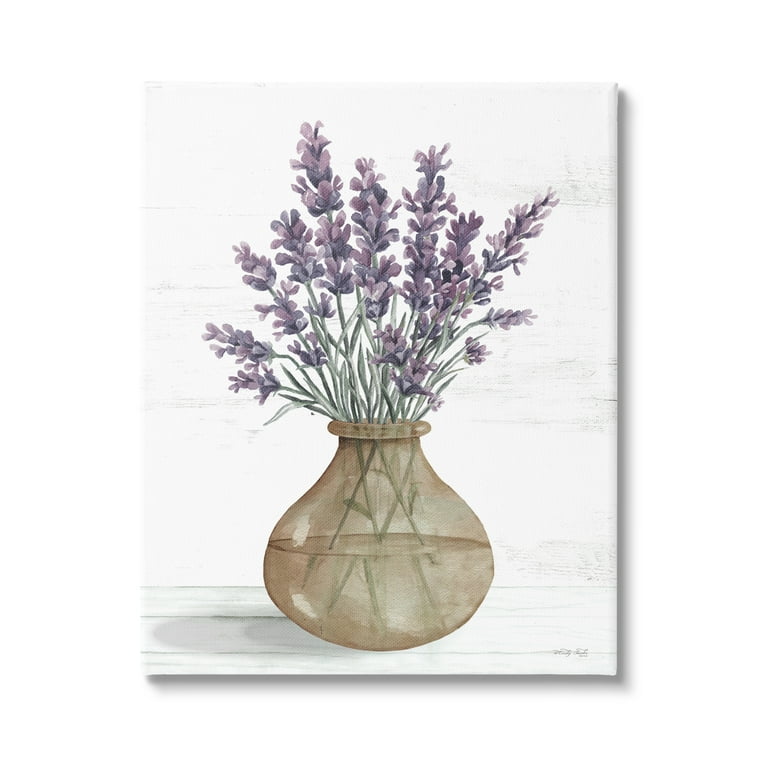The image depicts a hand-drawn painting on a white canvas, hanging unframed on a white wall. The painting features a translucent, light brown vase with a narrow neck, sitting on a painted wooden surface. The vase contains water filled up to halfway, allowing the viewer to see the green stems of the flowers inside. Emerging from the vase are multiple stems with dark green leaves and small purple flowers. The detailed artwork captures the delicate nature of the flowers and the subtle translucency of the water-filled vase. A shadow is visible on the bottom right side of the painting, and the artist's signature is also present in that corner, adding an authentic touch to the serene and minimalist composition.